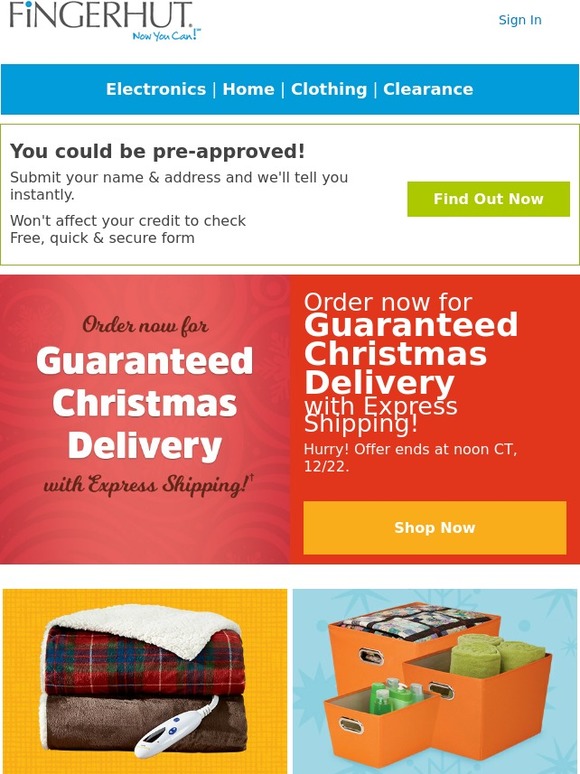The image features a screenshot of a website that closely resembles Fingerhut. At the top-left corner, the distinctive Fingerhut logo is prominently displayed, signaling the website's identity. Directly beneath the logo, a motivational tagline reads, "Now You Can!" written in blue font, complete with an enthusiastic exclamation point.

On the top-right corner, there is a simple "Sign In" link for users who wish to access their accounts. Below this link, a navigation bar offers various categories: "Electronics," "Home," "Clothing," "Clearance," providing quick access to different shopping sections on the site.

There is also a prominent information box that encourages users to apply for pre-approval. It states, "You can be pre-approved. Submit your name and address and we'll tell you instantly. Won't affect your credit to check. Free, quick, and secure form."

Additionally, situated on the left side of the page, a bright lime green button labeled "Find Out Now" invites users to initiate the pre-approval process, emphasizing the ease and immediacy of the service provided.